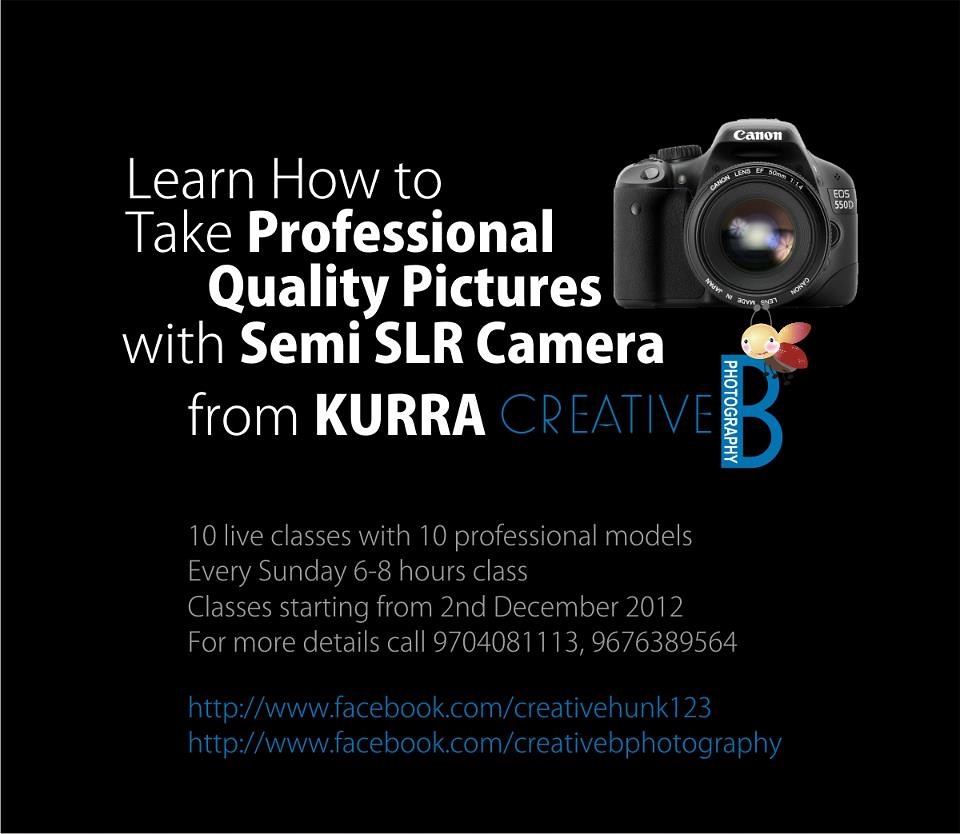The advertisement, set against a square black background, promotes a photography course titled "Learn How to Take Professional Quality Pictures with Semi-SLR Camera" offered by Cura Creative. The text details that the course consists of 10 live classes, each featuring a different professional model, held every Sunday with sessions lasting from 6 to 8 hours. Classes commence on December 2nd, 2012. For inquiries, the contact numbers provided are 970-408-1113 and 967-638-9564. The ad also includes two Facebook URLs: facebook.com/creativejunk123 and facebook.com/creativebphotography. In the upper right corner of the image, there’s a Canon camera embellished with a charming bee character. The bee has a yellow face, pink-yellow-maroon wings, a brown body, and black legs, adding a whimsical touch to the otherwise professional design.